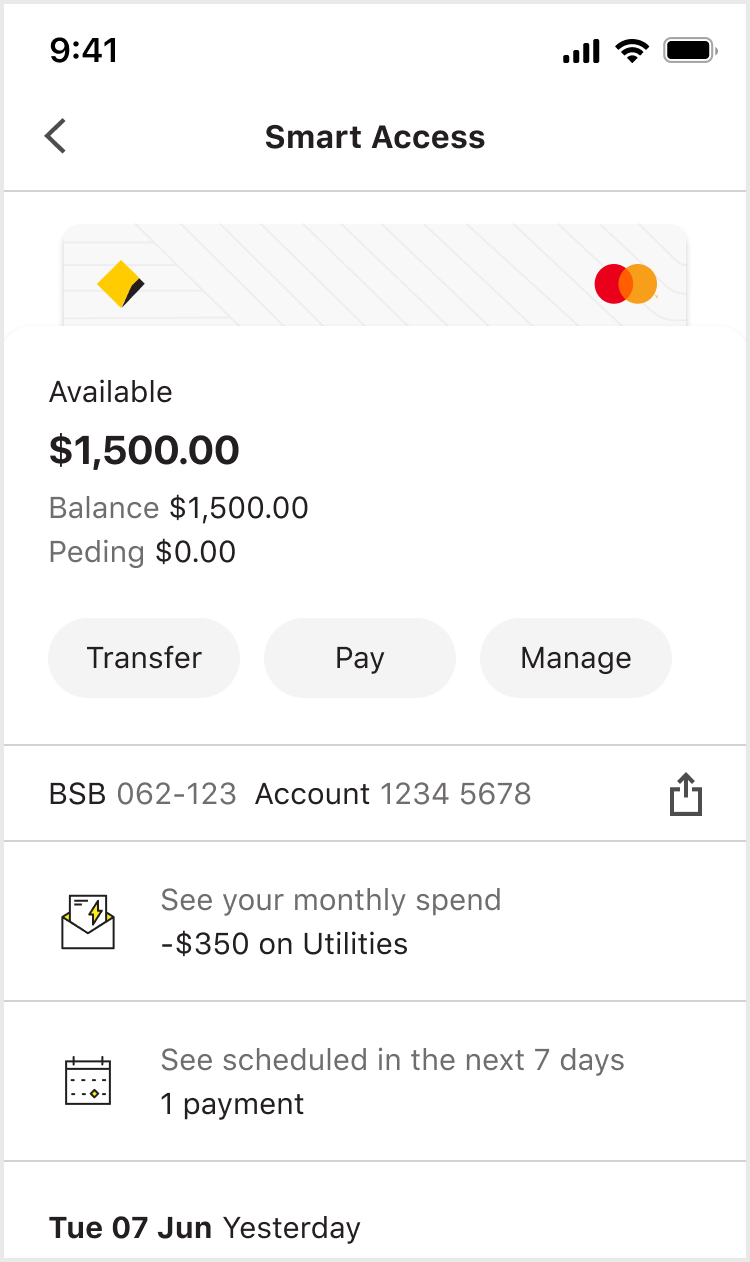A detailed and descriptive caption for the image could be:

The image depicts a smartphone screen on a white background, outlined by a thin, light gray line. At the top, the screen displays the title "Smart Access," followed by a horizontal gray bar. The bar features the MasterCard logo on the right and a tilted yellow square with a black edge on the left. Beneath the gray bar, the word "Available" is written in black letters, followed by a bold black amount of "$1500." In light gray, the word "Balance" appears with the corresponding amount "$1500." Below, "P-E-D-I-N-G," possibly meant to represent "Pending," displays with a balance of "$0" in light gray.

Further down, there are three elliptical buttons labeled "Transfer," "Pay," and "Manage" in medium gray, each centered within a light gray racetrack-shaped ellipse. A faint gray line below these buttons is followed by the text "B-S-B 062123 Account 12345678," with an upload icon to its right. Another thin gray line separates this row from the next section.

This next section features a money and wallet icon on the left, with the phrase "see your monthly spend" in light gray beside it. Below, it reads "$-350 on utilities" in medium gray. Following another light gray line, the icon of a calendar appears, with the text "see scheduled" and "next seven days" in light gray to its right. Underneath, the medium gray text reads "1 in payment."

The final section ends with "T-U-E 07 J-U-N" in bold letters, indicating the date "Tuesday 07 June" with "Yesterday" next to it.